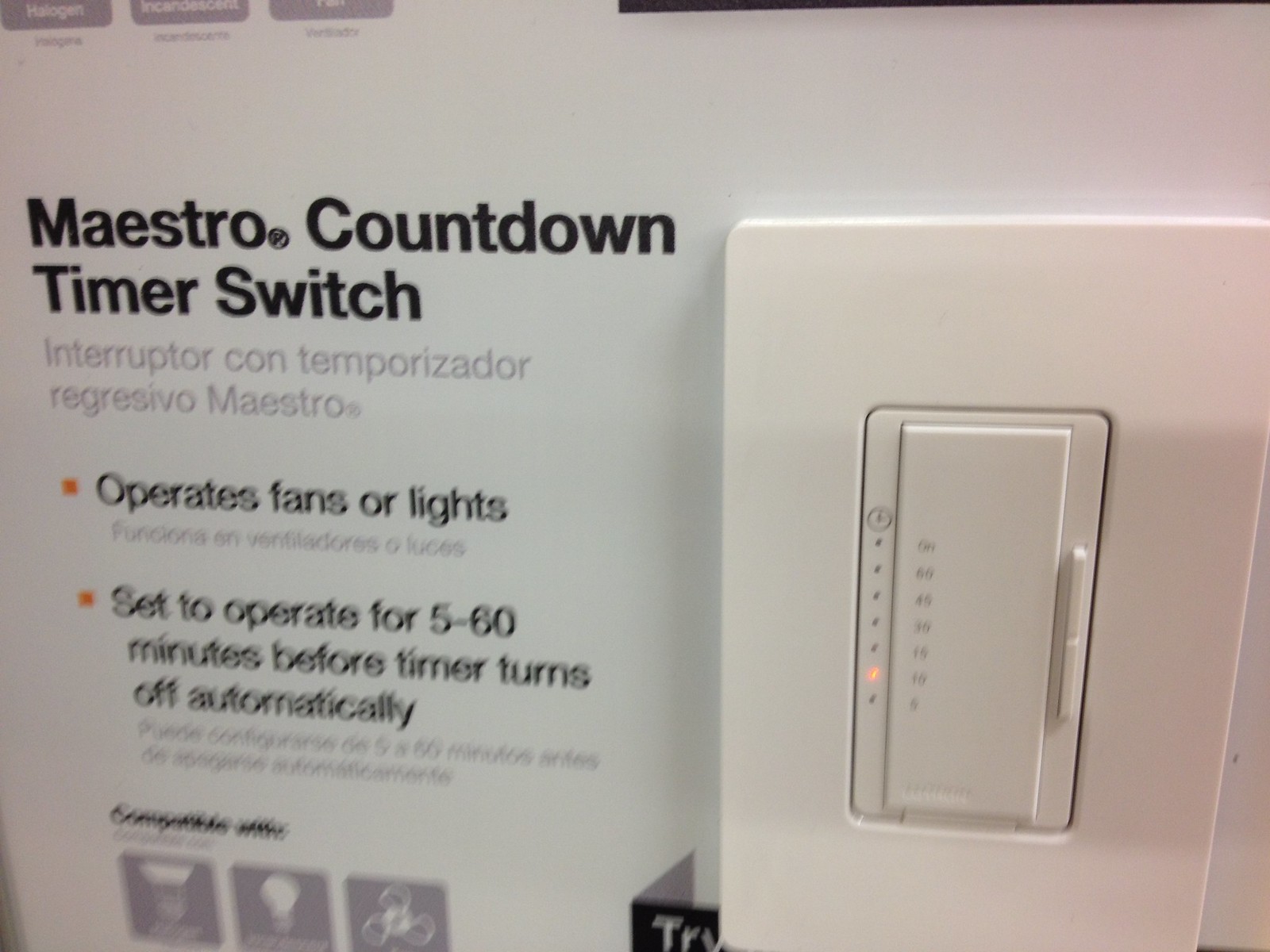The image is a detailed photograph depicting a packaged Maestro Countdown Timer Switch alongside the actual timer device. 

The packaging features a clean, white background with predominantly black or gray text. The primary text reads, "Maestro Countdown Timer Switch," accompanied by its Spanish translation, "Interruptor Contemporizador Regresivo Maestro." The front of the package includes two orange-bulleted lists detailing the timer's functions. The first bullet point states, "Operates Fans or Lights," and beneath it, the Spanish equivalent. The second bullet point reads, "Set to operate for 5 to 60 minutes before the timer turns off automatically," followed again by the Spanish translation.

At the bottom of the packaging, additional text indicates compatibility, showcased through small icons: a light bulb representing lights, a fan for fans, and an unclear first icon, likely representing electrical compatibility.

Next to the package is the actual Maestro Countdown Timer Switch, which is a rectangular white device. In its center is a smaller, door-like rectangle. The device features a vertical sequence of numbers, marked in ascending order from 5, 10, 15, 30, 45, and 60 minutes, with an "on" option at the top. Currently, an orange light is illuminated next to the "10" minute mark, indicating the active timer setting.